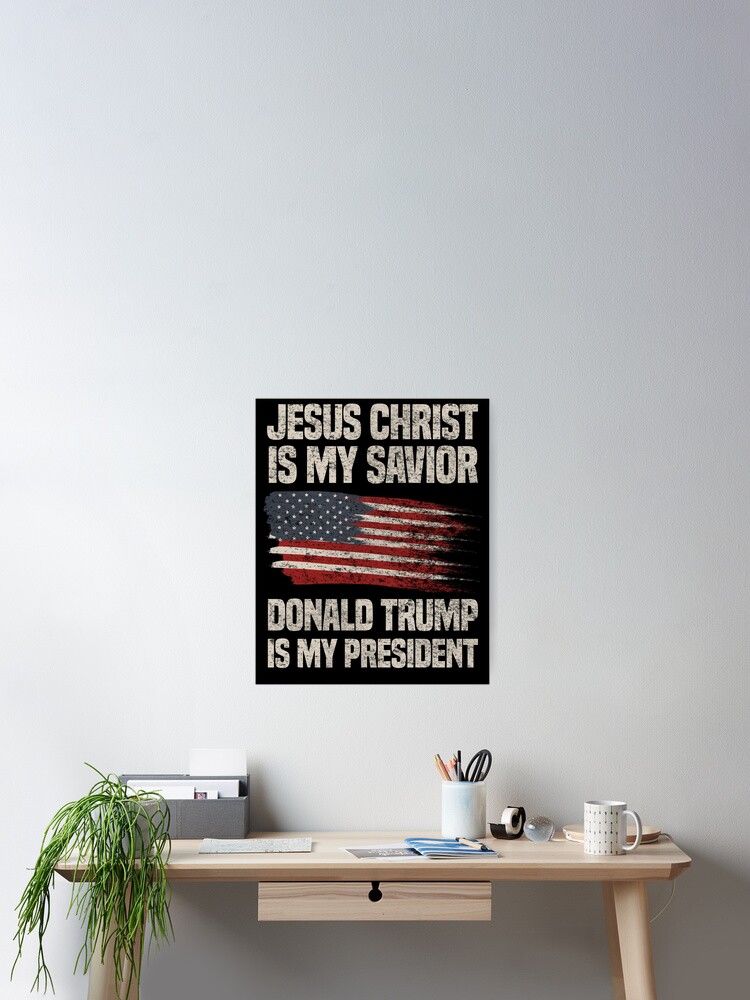The photograph is a vertically rectangular, full-color, staged indoor image featuring a light gray wall as the background with a washed-out effect on the left side, suggesting light from the other side. At the bottom of the frame is a light wooden desk with a single pull-out drawer in the center. On the left corner of the desk is a green plant, while on the right side, there's a white cylindrical desk lamp with an L-shaped arm, accompanied by a white coffee cup. Between the plant and lamp, there is a cylindrical container holding pencils and possibly scissors, along with a roll of tape. Above the desk hangs a black square poster, centered slightly to the left, featuring the American flag and the text: "Jesus Christ is my Savior, Donald Trump is my President." The colors in the scene include shades of tan, green, white, black, red, blue, and gray.